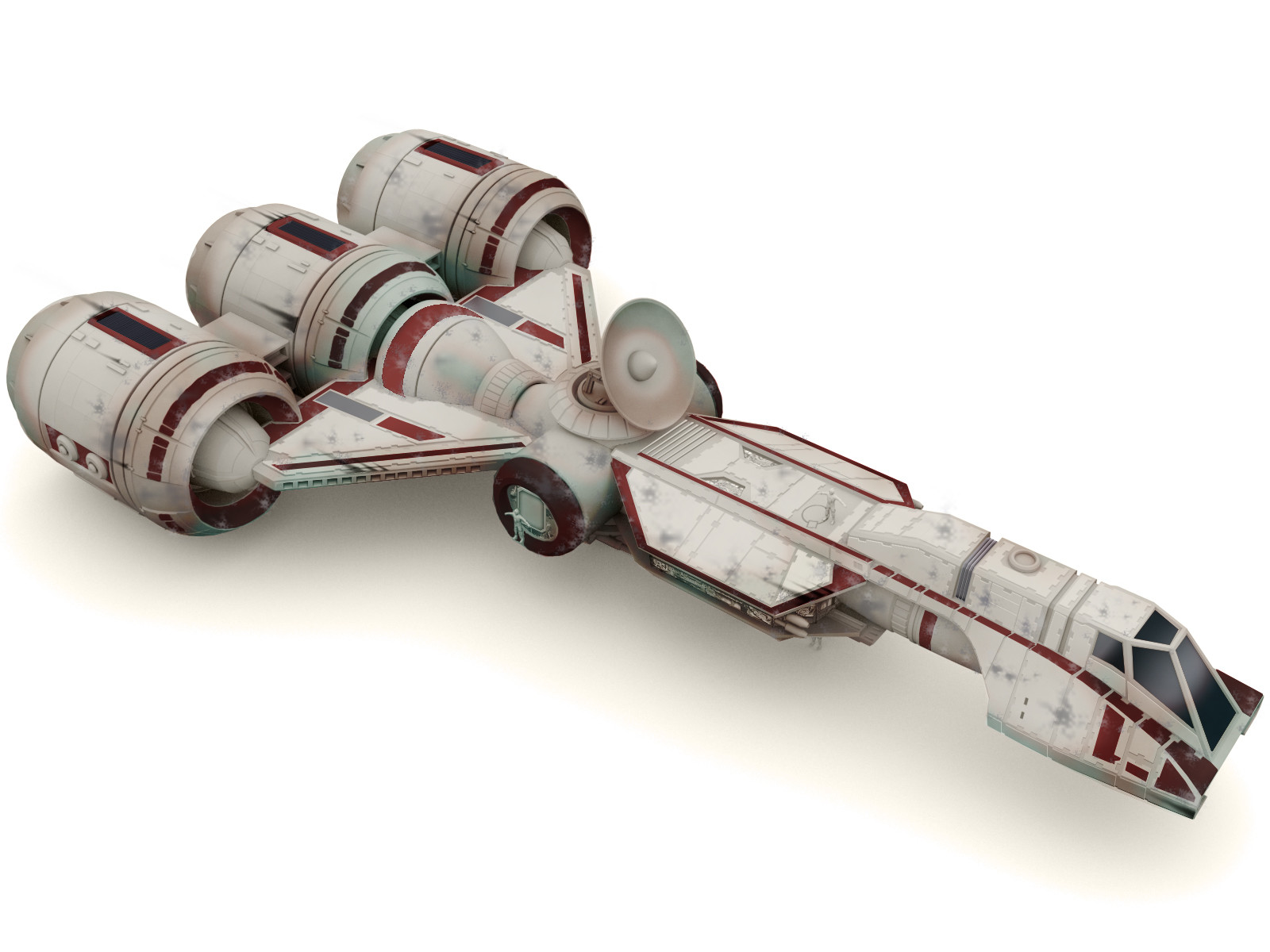This image depicts a detailed model of a spacecraft, likely from the Star Wars universe, specifically the Corellian Courier. The spacecraft is predominantly white, adorned with red and maroon-colored markings and rusty brown details that suggest wear and age. It features three large engines positioned at the back, oriented towards the top left of the image, with a long body extending to the bottom right. The middle engine connects to the main structure of the ship, giving it a distinctive T-shape when viewed from above. The front of the spacecraft includes black windows, and a satellite dish is visible on the top. The background is plain white, devoid of text or other distractions, focusing entirely on the spacecraft model. The picture does not indicate whether it was taken indoors or outdoors or the time of day it was captured, but the smudges and worn detailing enhance its realistic, rugged appearance.